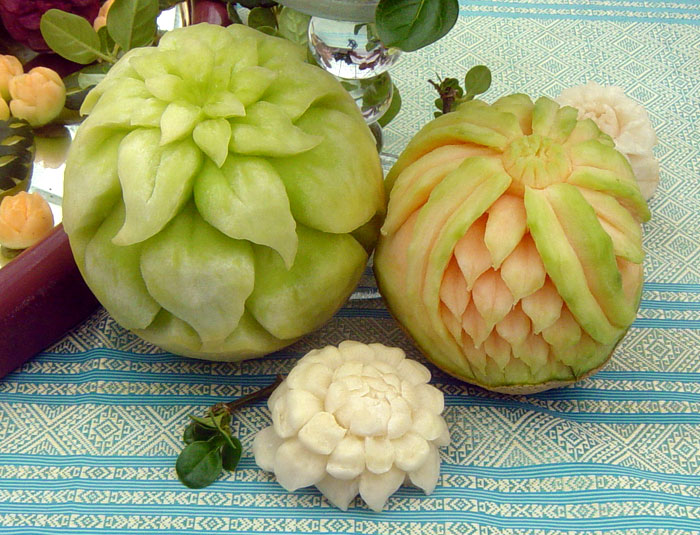The image is a color photograph in landscape orientation showcasing three meticulously crafted fruit sculptures. The primary subjects are the two large, round melons positioned near the top of the image. The melon on the top left is a light green honeydew with intricately carved leaves creating a blossom pattern. The top right melon features a similar floral carving but with a light green exterior and cream-colored petals. At the bottom center of the image is a smaller, white flower carved from what appears to be a different type of melon, possibly a cantaloupe. The fruit sculptures are artistically arranged on a tabletop covered with an aqua blue and white striped tablecloth. Additional small floral decorations made from food and green leaves can be seen in the upper left corner. In the background, faint reflections suggest the presence of a glass or crystal object, adding to the elegant presentation of the scene.